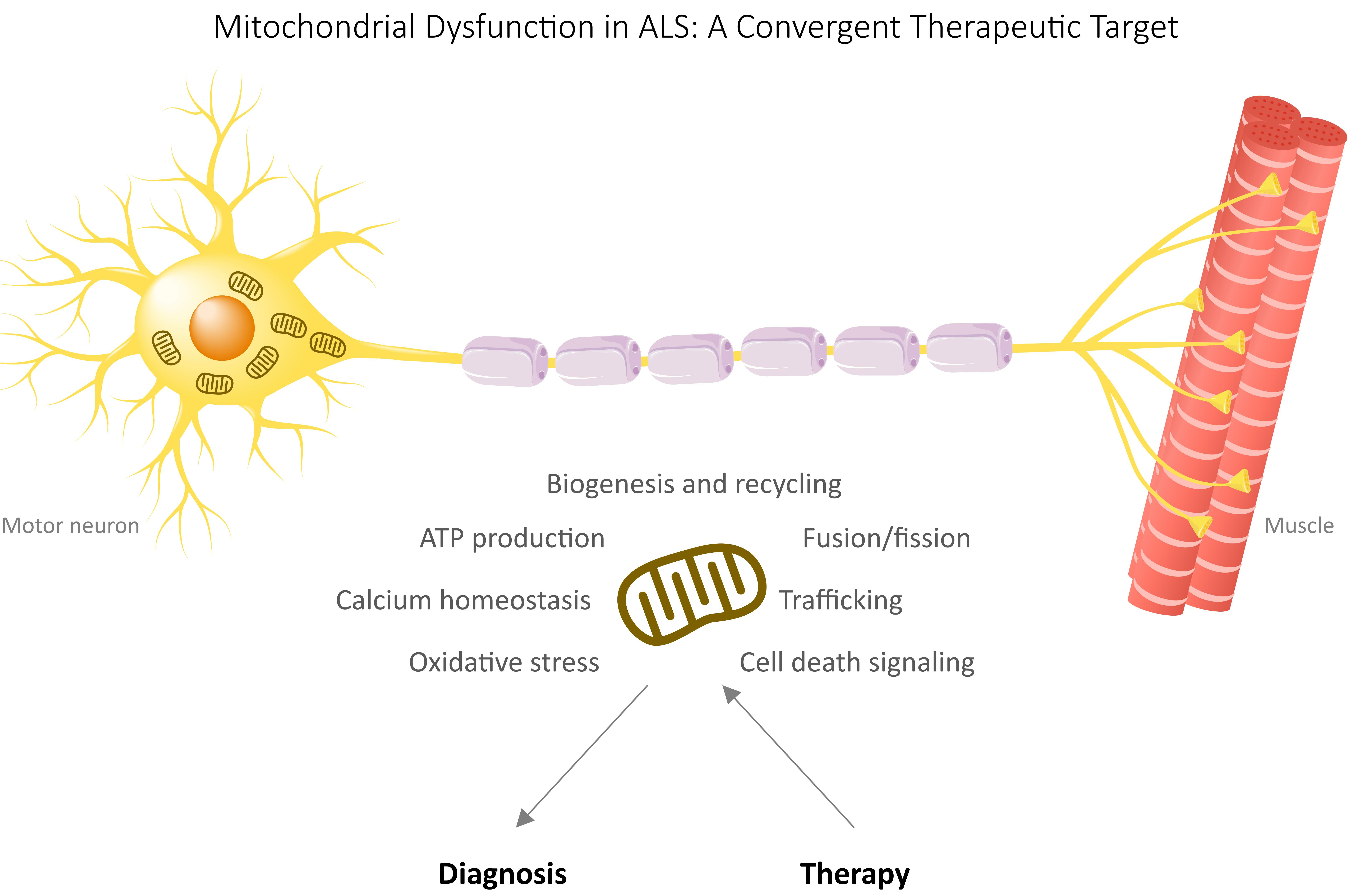The image resembles a detailed diagram from a biology or medical textbook, titled "Mitochondrial Dysfunction in ALS: A Convergent Therapeutic Target." The central focus is a yellow motor neuron depicted with roots extending from it, leading into a long yellow strand, presumably the axon, adorned with white, milk-jug-like structures representing myelin sheaths. Further along, this axon branches into multiple strands that connect to three pink, striped tubular structures labeled as muscle fibers. These muscle fibers are depicted with a pinkish-white color, somewhat reminiscent of curled yoga mats. The diagram includes numerous labels for various cellular processes and components, such as "biogenesis and recycling," "ATP production," "calcium homeostasis," "oxidative stress," "fusion and fission," "trafficking," "cell death signaling," "therapy," and "diagnosis," each indicated with corresponding arrows. All of these elements are set against a white background, providing clarity to the detailed biological mechanisms being illustrated.